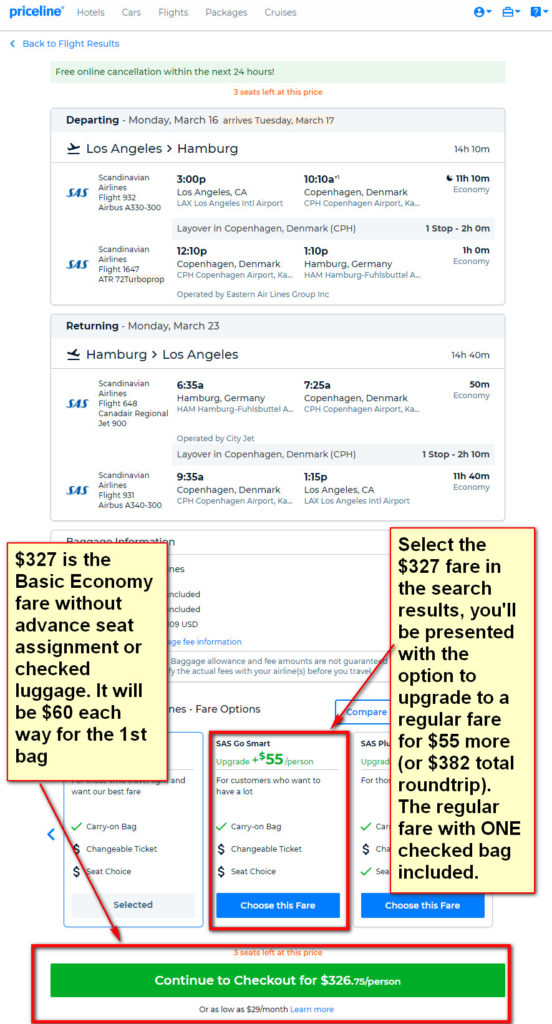A screenshot of a flight itinerary is displayed on a webpage from a travel service company, identified by the Pricelinem logo in the top left corner. The header menu of the site includes options for "Hotels," "Cars," "Flights," "Packages," and "Cruises." Below this, the flight itinerary details a round trip departing from Los Angeles to Hamburg and returning from Hamburg to Los Angeles, though the text for the specific flight details is too small and blurry to read.

Further down the page, there is a tan-colored rectangular box with a red border, displaying the fare of $327. This fare is for a basic economy ticket, which does not include an advanced seat assignment or checked luggage. An additional fee of $60 each way is required for the first checked bag. An arrow points to a green rectangular button at the bottom of the image, which is highlighted with a red border and reads "Continue to Checkout for $326." To the right of this button, another tan-colored box is visible, though its contents are not specified.